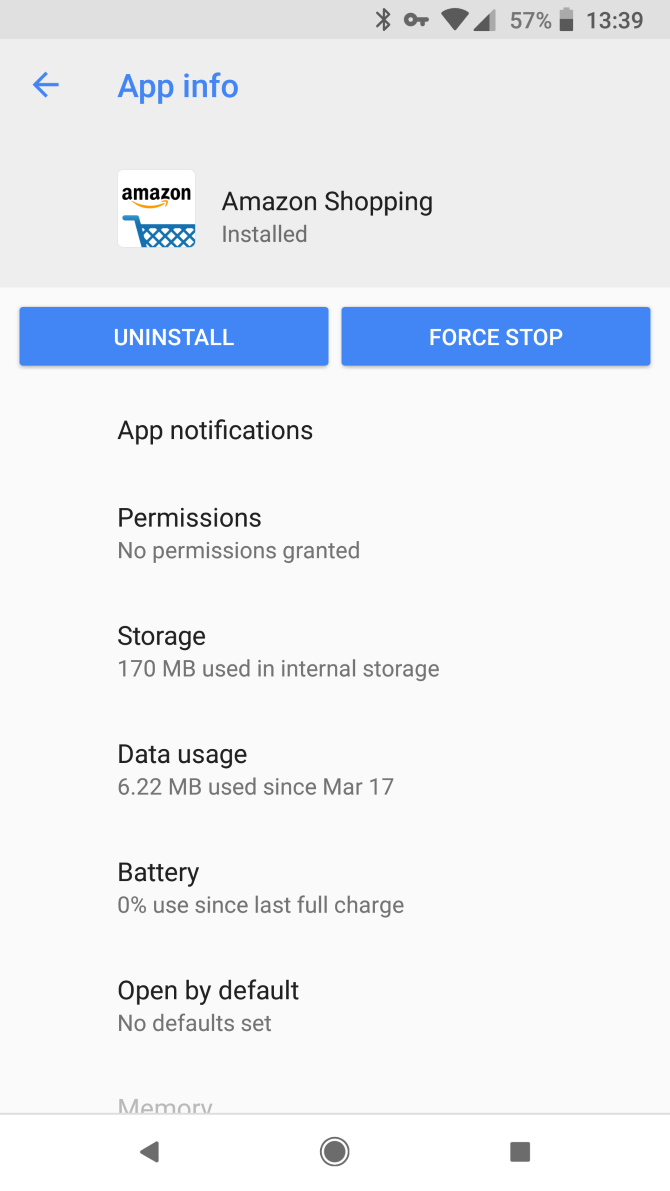The image depicts a smartphone screen displaying the "App Info" page for the Amazon Shopping app. At the top, the status bar shows various icons, including the Bluetooth symbol, a key icon, and other indicators, with the battery level at 57%. The time displayed is 13:39, indicating 1:39 PM in military time.

The main section of the screen shows the "App Info" heading in blue, followed by the Amazon logo and the label "Amazon Shopping." The user is likely in the settings or app management section, as options to "Uninstall" or "Force Stop" the app are visible. Below these options are several categories:

- **App Notifications**
- **Permissions**: Indicates "No Permissions Granted."
- **Storage**: Shows "170 MB used in internal storage."
- **Data Usage**: Displays "6.22 MB used since March 17th."
- **Battery**: Reports "0% used since last full charge."
- **Open by Default**: Notes "No Default Set."
- **Memory**: This category is partially visible but does not show specific details.

Beneath these categories, the screen shows icons resembling play, stop, and record buttons.